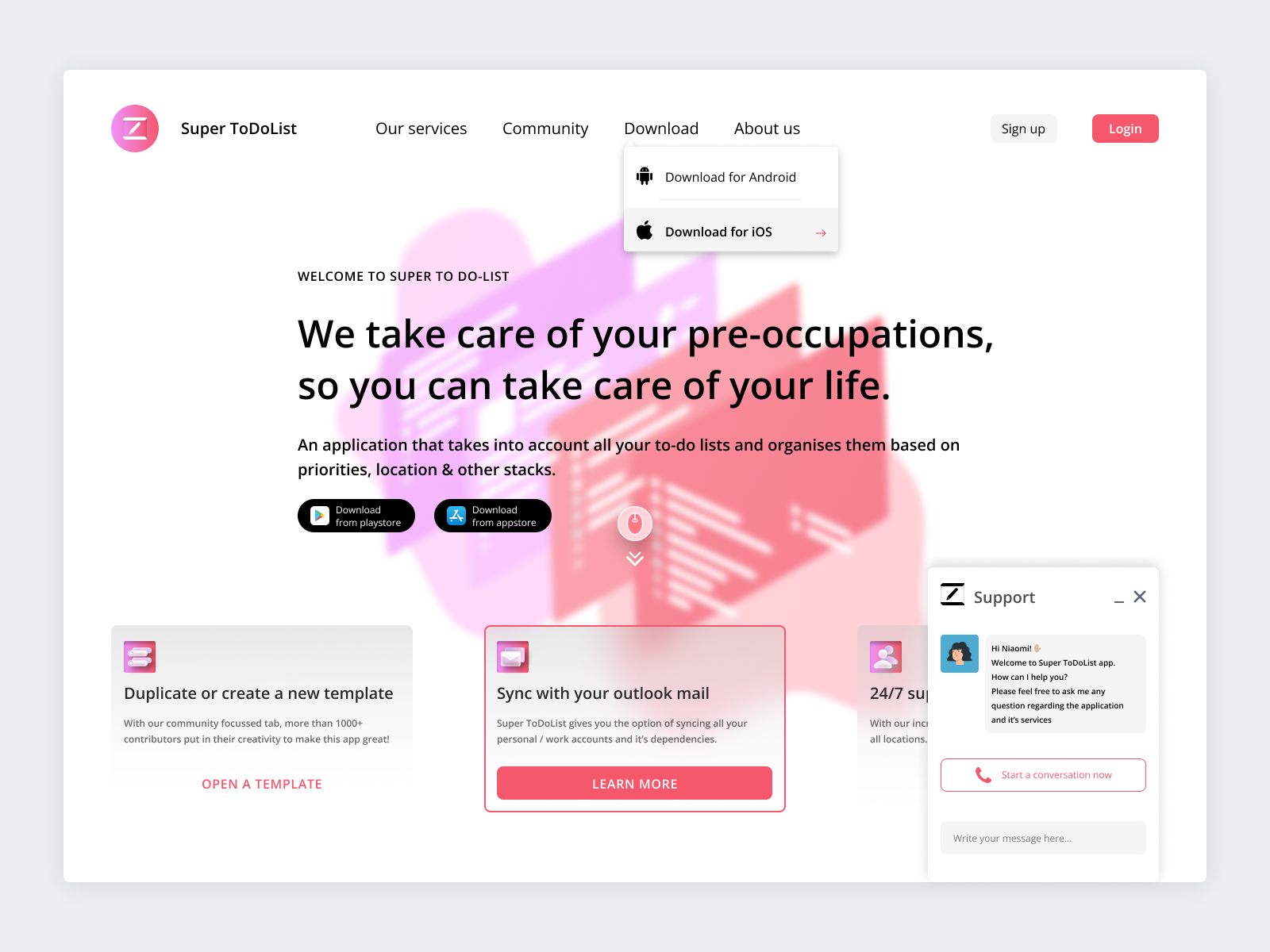On the homepage of the "Super To-Do List" website, the layout and features are meticulously arranged against a white background outlined in gray. On the left side, a navigation panel features a pink circle with a white "C" in the center, followed by menu items labeled "Our Services," "Community," "Download," and "About Us" in black text. Below this section, a banner, somewhat hidden under the "Download" and "About Us" tabs, shows a black alien icon with the text "Download for Android," followed by another banner featuring a black Apple icon labeled "Download for iOS."

On the right side, there is a slim gray banner with the text "Sign Up" in black, and next to it, a pink banner with "Log In" in white. In the middle of the page, the heading "Welcome to Super To-Do List" is prominently displayed, accompanied by the tagline "We take care of your preoccupation so you can take care of your life." Below this, a brief description highlights the app's functionality: it prioritizes and organizes to-do lists based on various factors such as priorities and locations.

Two black banners are centered beneath the welcoming text, providing download links for different platforms: "Download from Play Store" with the Google Play Store icon, and "Download from App Store" with the iOS icon. Further down, two gray-shaded banners provide additional options. The first banner, shaded in gray, reads: "Duplicate or create a new template," highlighting the app's community focus, which boasts over 1,000 contributors. It includes a pink "Open a Template" button. The second gray box, outlined in pink, offers a syncing feature: "Sync with your Out mail. Super to-do list gives you the option of syncing all of your personal and work accounts and its dependencies." A blue or pink banner with "Learn More" in white is also present.

To the right again, another banner indicates "24/7 support," but it becomes partially obscured by a popup message. The white popup, titled "Support," warmly greets the user: "Hi Naomi, welcome to Super To-Do List app. How can I help you? Please feel free to ask me any questions regarding the application and its services." The dialog box is complemented by a pink banner with "Start a Conversation Now" and a small pink phone icon. This support message includes a gray banner where users can type their inquiries directly into the provided space.